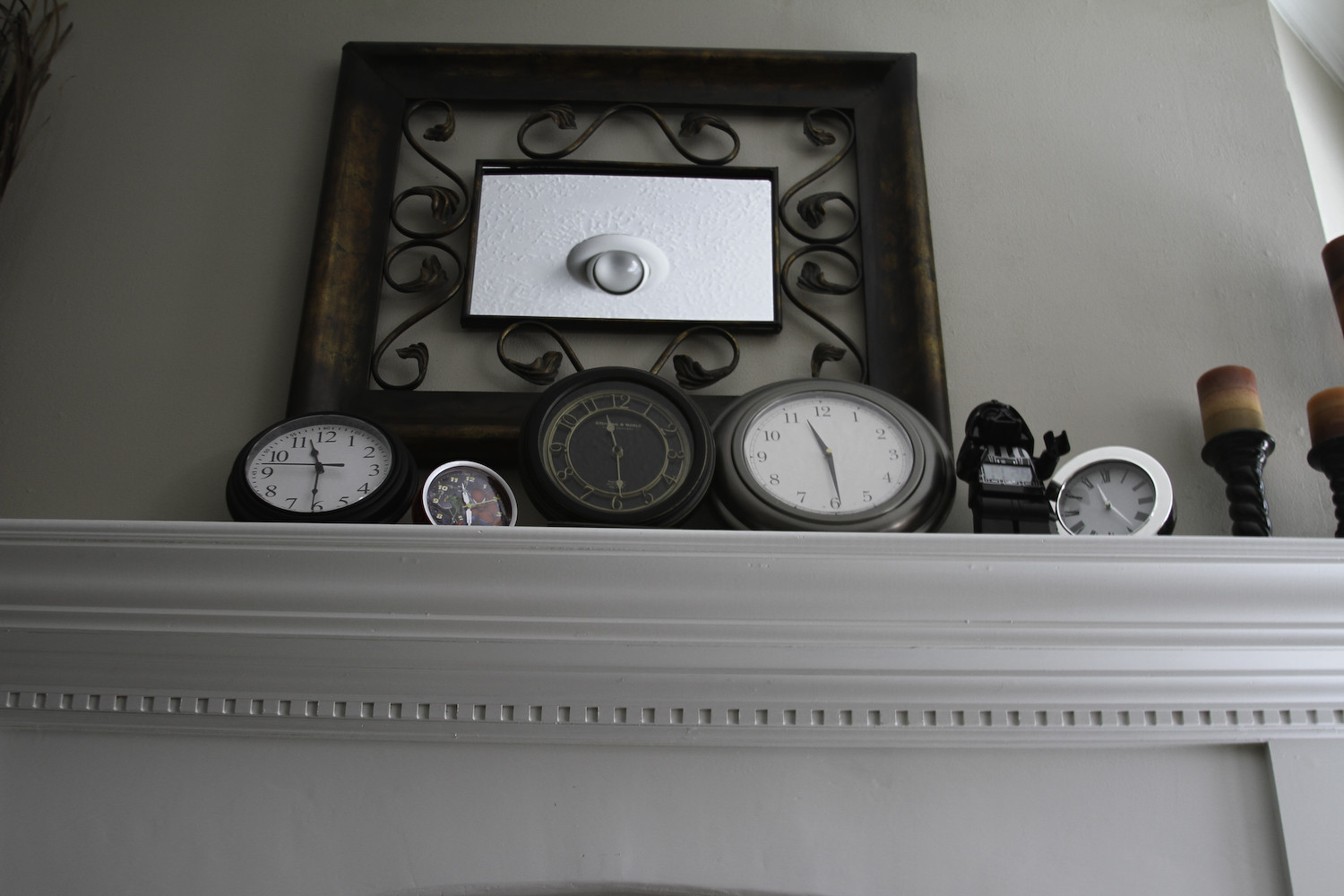This indoor photograph captures the intricate details of a stylish mantle, viewed from floor level, adorned with a variety of unique clocks and decor. The mantle, matching the medium to light gray walls, features a sophisticated edging pattern of alternating deep and raised squares. 

From left to right, the mantle showcases an array of clocks: a round clock with a white face and black trim, a small black and silver clock, an ornate black and gold clock, and another black clock with a white face. Among these timepieces, a robot-shaped clock with its belly as the time display adds a quirky touch. Toward the right, a silver clock with a white face sits beside two elegant candle holders with black candlesticks.

Dominating the space above the mantle is a rectangular frame with intricate black scrollwork encasing what seems to be an image of a ceiling light with a clear lens, almost resembling an eye. This framed artwork is set in a dark brown frame, creating a striking focal point. The collective display of clocks presents a mix of black, white, and pewter frames, with several clocks showing the time as 11:26, enhancing the scene's eclectic charm.